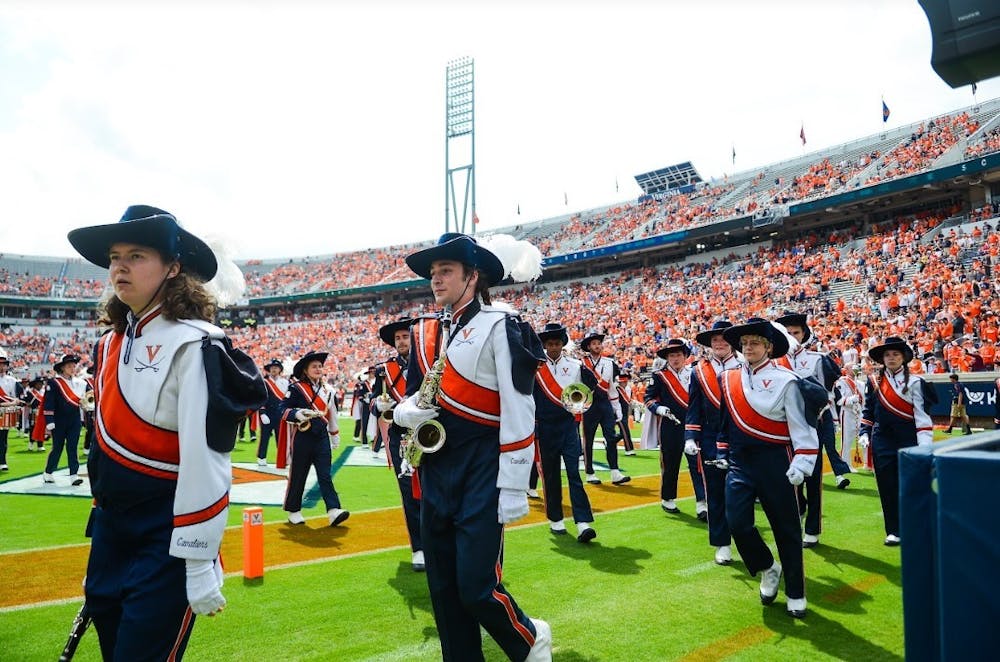The photograph captures a vibrant scene during a football halftime show featuring a meticulously organized marching band, all attired in striking uniforms. Each band member sports blue pants with red stripes running down the sides, paired with white jacket tunics that boast sharp, angular elbows and shoulders. A distinctive red sash with a central white stripe stretches diagonally across their chests. Their uniforms are further detailed with asymmetrical design: the left shoulder and left sleeve are white with a red stripe, while the right shoulder and right sleeve are blue. Completing their ensemble are black, large-brimmed cowboy hats adorned with white feather boas, alongside white shoes.

They stand on a football field covered in short, bright green artificial grass, interspersed with various brown and white areas that demarcate the field lines and zones of play. Surrounding the field are the step-like bleacher seating, fully populated with an audience primarily dressed in orange, indicating a high level of enthusiasm and support for the event. Towering in the background are prominent floodlights, although unlit, suggesting it is daytime, as evidenced by the clear, sunlit sky.

The scene also includes various band members holding different musical instruments such as trumpets, adding to the dynamic atmosphere. Both young men and women participate in the performance, unified in their elaborate and colorful attire, contributing to the lively and spirited halftime show.